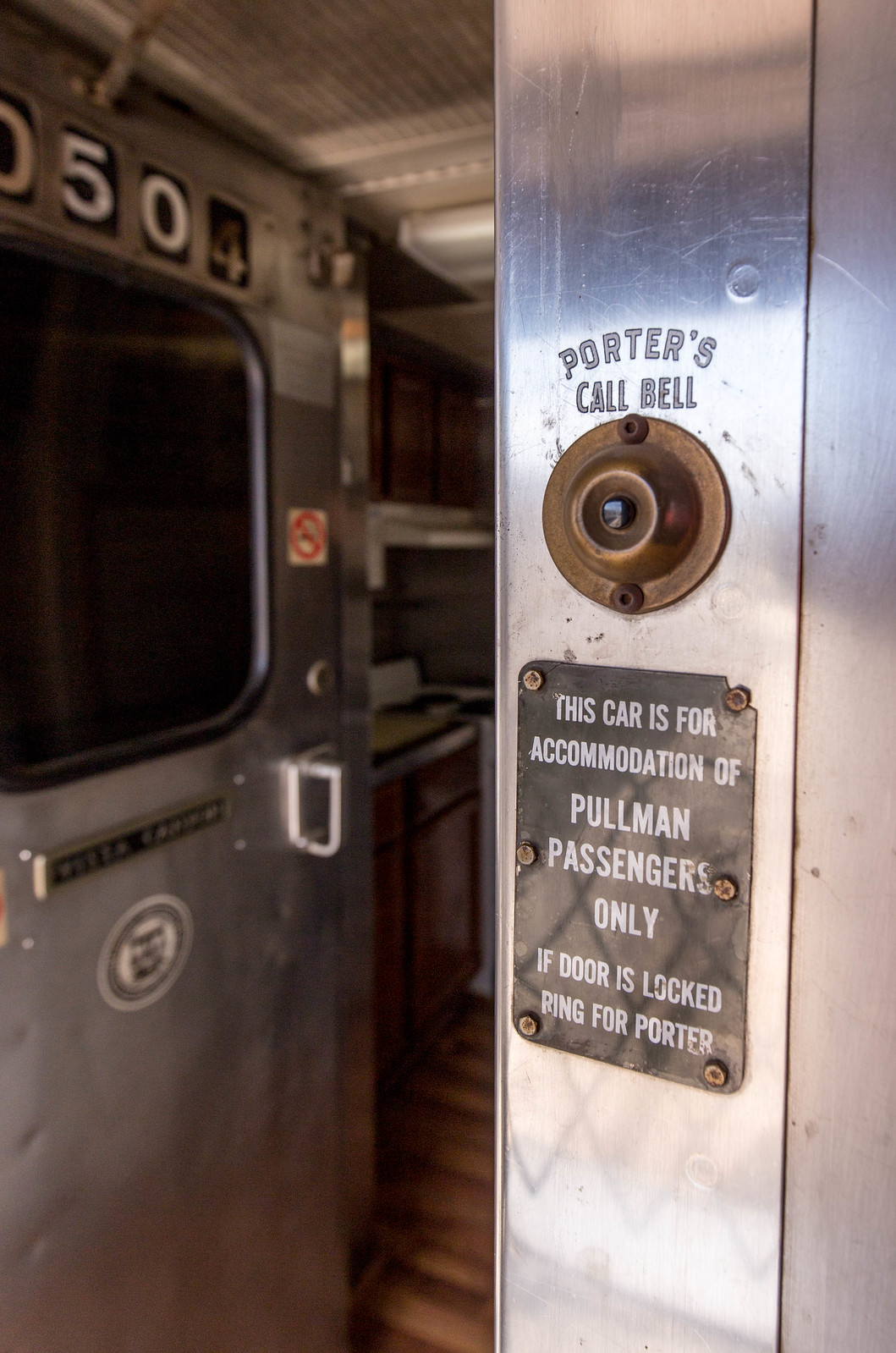The photograph showcases the interior of a train car, focusing on a stainless steel area adorned with various noticeable features. To the very right, there is a prominent, shiny, yet marked, textured surface that contains the embossed lettering "Porter's Call Bell." Directly beneath this engraving is a bronze-colored bell, attached to a black placard that is bolted onto the steel wall with six screws. The placard displays white instructions, reading: "This car is for accommodation of Pullman passengers only. If door is locked, ring for Porter." Moving left, the train car continues with stainless steel surfaces, and more than halfway across the image, a door marked with the number "050" comes into view. Near the back of the car, a window is noticeable, adding to the sleek yet industrial aesthetic of this Pullman train interior.